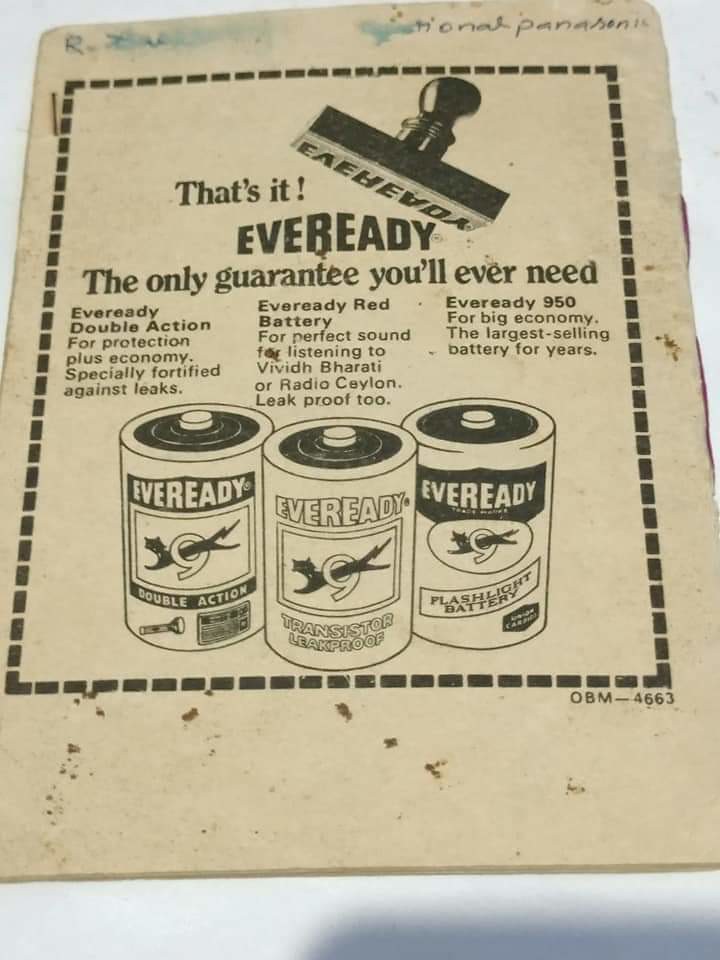This photograph showcases a vintage advertisement on yellowed, water-damaged paper, likely from an old magazine or newspaper. A rectangle with dashed lines, indicating it could be cut out as a coupon, frames the ad. The paper is stamped with the Ever Ready logo at the top, which appears to have been applied using a rubber stamper that left an ink mark resembling a cat jumping through a number nine. Below the stamp, bold text proclaims, "Ever Ready, the only guarantee you'll ever need."

Further down, the advertisement elaborates on the benefits of Ever Ready batteries in three columns:

1. "Ever Ready Double Action: For protection plus economy, specially fortified against leaks."
2. "Ever Ready Red Battery: For perfect sound for listening to VIVIDH BHARATI or Radio Ceylon, leak-proof too."
3. "Ever Ready 950: For big economy, the largest selling battery for years."

At the bottom, black-and-white illustrations depict three batteries side by side, labeled "Double Action," "Transistor Leak-Proof," and "Flashlight Battery," each adorned with the Ever Ready logo. An old staple is visible at the side, suggesting it was once bound in a publication. The handwriting at the top of the page is faded, contributing to the paper's aged appearance.